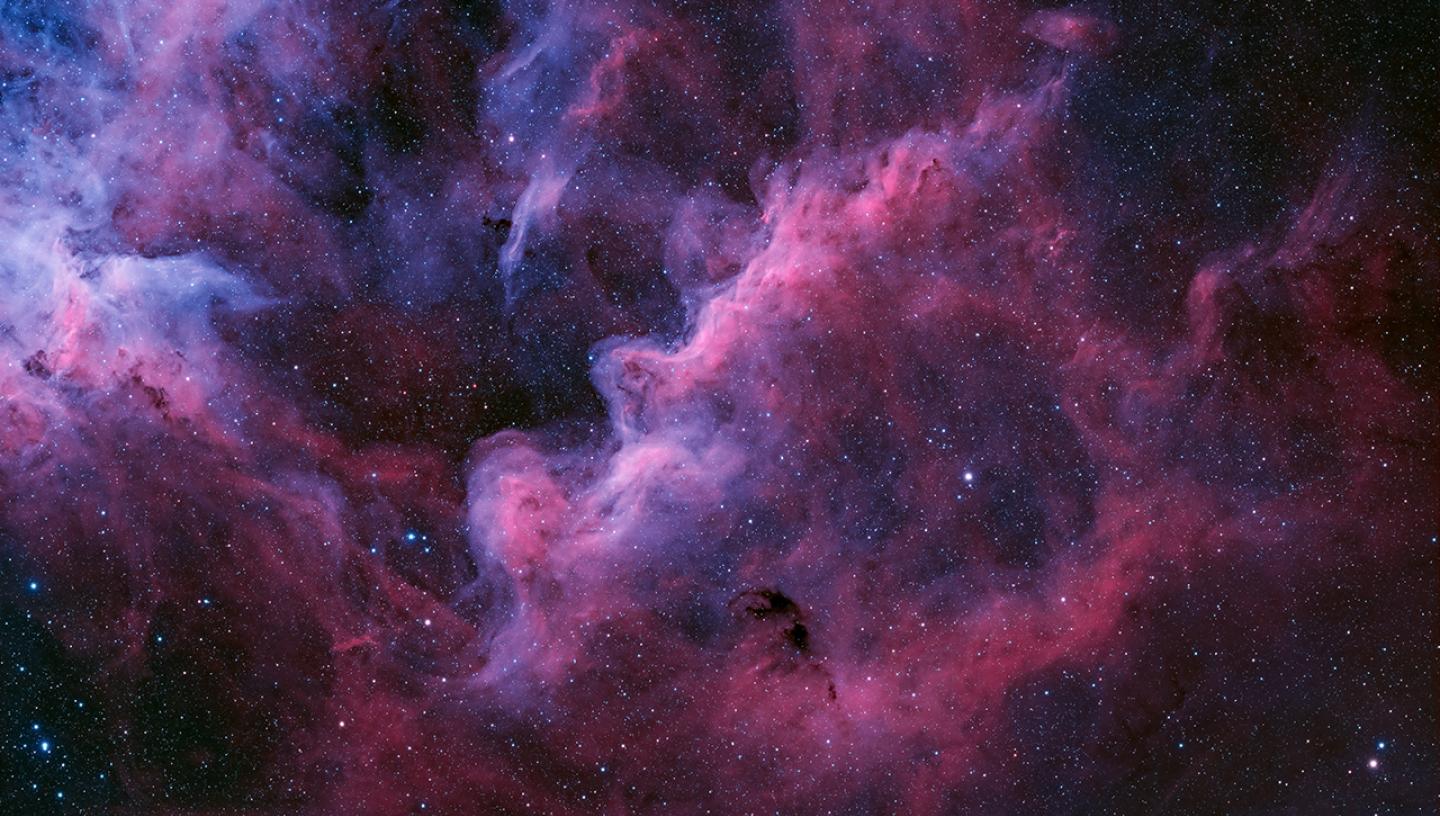This vibrant space art, presented in landscape orientation, showcases a stunning star nebula depicted in an enhanced photographic style with special color filters. Dominated by billowy clouds of gas in striking shades of pink and white, the nebula fills the majority of the image. These luminous clouds blend seamlessly with interspersed blues, creating a dynamic and ethereal scene. Thousands of stars punctuate the composition, with concentrations in the top right, bottom, and left bottom quadrants, allowing the cosmos to gleam through the gas clouds. A particularly bright star emerges from the nebula on the right, distinctively shaped like a horse's head in profile. The dark black star field frames the nebula, adding depth and contrast to this entrancing, color-saturated portrayal of outer space.